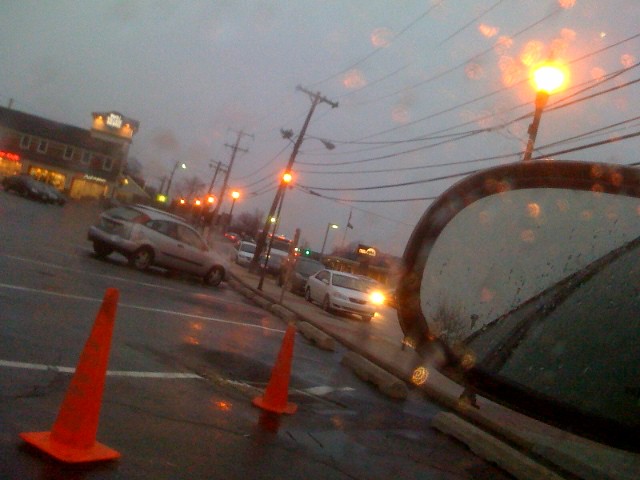The image captures a bustling parking lot filled with various parked cars, framed by two bright orange construction cones. Rain-soaked pavement and droplets hint at an ongoing drizzle, adding a reflective sheen to the scene. Several more vehicles are visible on the adjacent street, surrounded by an array of businesses, including a prominently displayed Pizza Hut sign among other restaurants. In the corner of the image, a black side mirror suggests the perspective of someone seated in a nearby car. Overhead, a network of power lines crisscrosses the sky, interspersed with street lights, while a green traffic light in the distance signals the steady flow of traffic. Despite the rainy weather, the area appears lively and well-frequented.